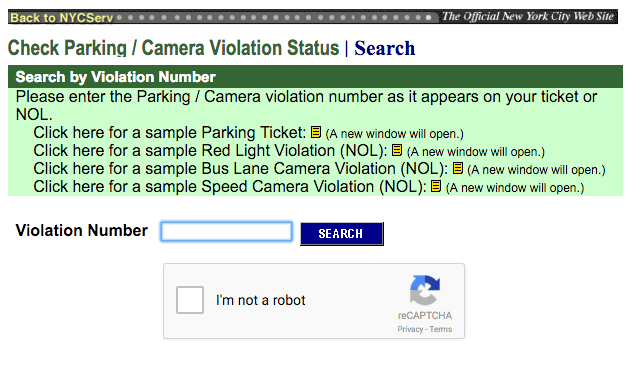The image is a screenshot of a website designed for checking parking and camera violations in New York City. At the very top of the page is a narrow gray header. On the upper left corner of this header, written in yellow font, it says "Back to NYC SERB." On the upper right corner, written in white font, it reads "The Official New York City Website."

Below this header, the background turns white. On the left side, in gray font, it says "Check Parking / Camera Violation Status," followed by a vertical line. To the right of this, in blue font, it says "Search."

Further down, there's a green horizontal border. Within this green section, written in white font, it says "Search by Violation Number." In this green segment, black font instructions read, "Please enter the parking/camera violation number as it appears on your ticket or NOL," providing guidance for users.

The lower part of the website has a white background. Below the light green section, there is a space labeled "Violation Number" accompanied by a search box. Adjacent to the search box is a blue button with the word "Search" written in white font. Centered below this search area is the familiar "I'm not a robot" CAPTCHA checkbox, which users must click to proceed to the next page.